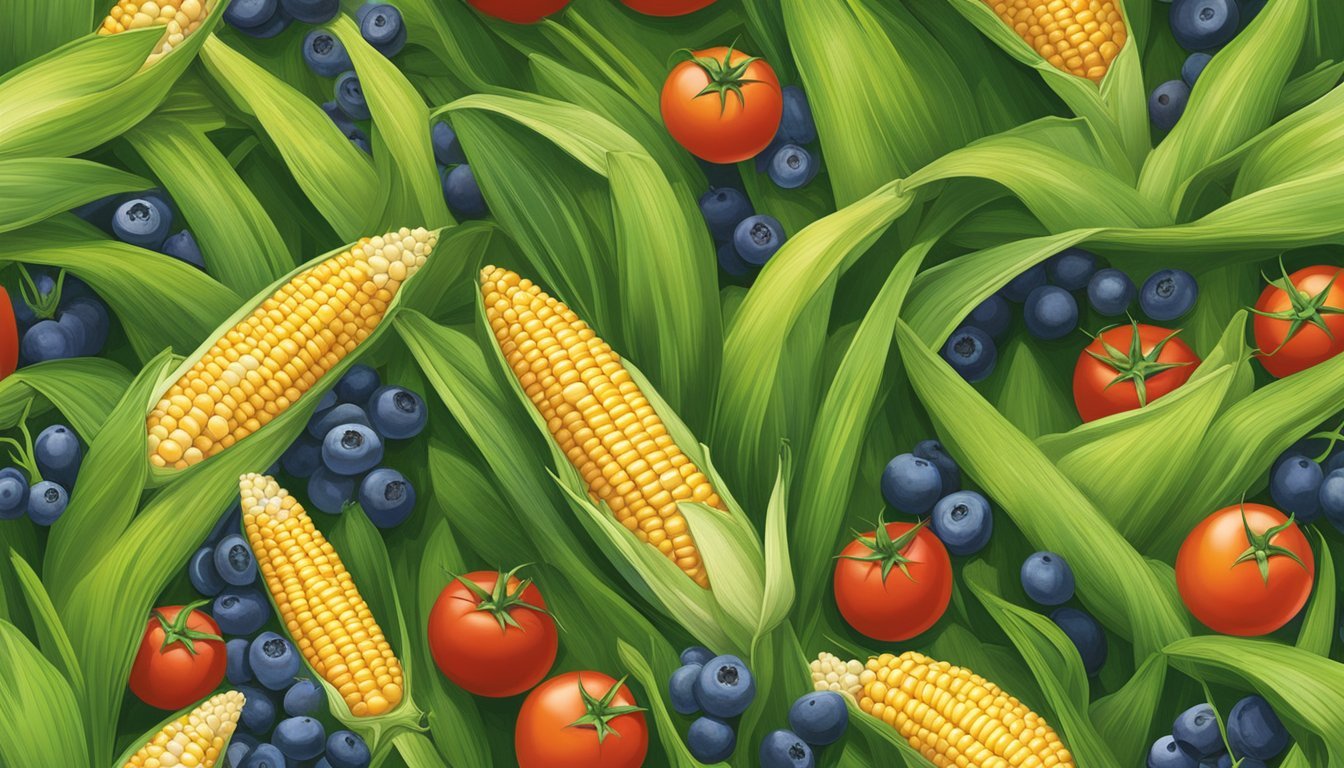The image is a beautifully detailed and colorful digital illustration showcasing a bountiful arrangement of corn, tomatoes, and blueberries. The dominant feature is the corn, with ears partially husked to reveal kernels that are predominantly yellow with a few white tips. The corn is nestled within green leaves that exhibit white striations and hints of gold. Interspersed among the corn are plump, hand-picked tomatoes, notable for still having their green stems attached. Adding further vibrancy and contrast are the numerous blueberries scattered throughout the scene. The composition is not just visually striking with the mix of yellow, green, red, and blue hues but also evokes a sense of freshly harvested produce, ready to be savored.